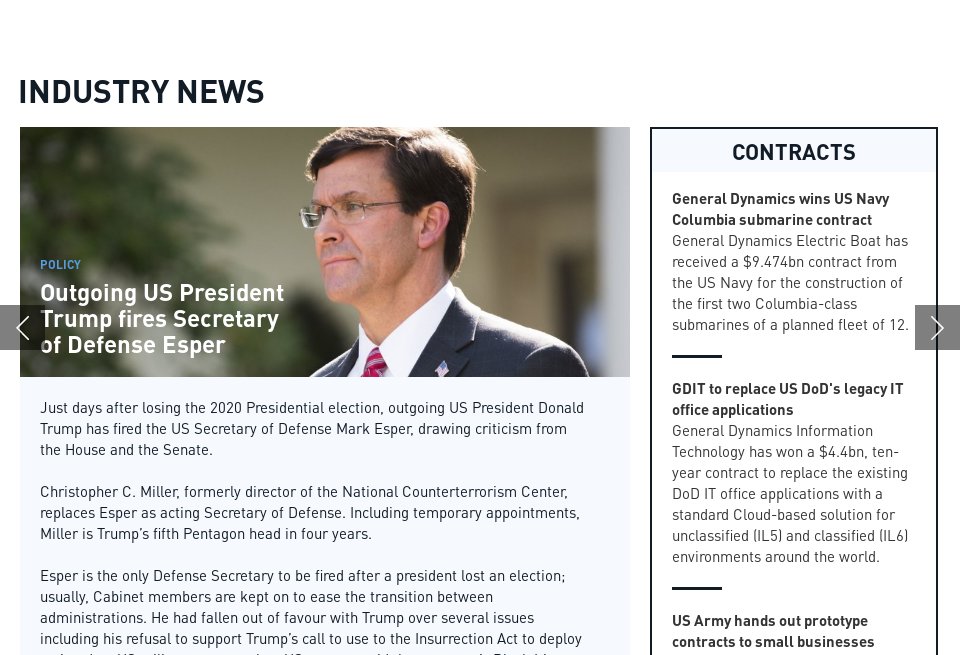The image appears to be a computer screenshot featuring a detailed news update related to industry news in the upper left-hand corner. There is a prominent photograph of a man with short black hair, wearing glasses, dressed in a black suit with a white shirt and red tie, looking to the left. Adjacent to his image, text reads: "Policy: Outgoing US President Trump Fires Secretary of Defense, Esper."

Beneath the headline, the news excerpt captures significant details: "Just days after losing the 2020 presidential election, outgoing US President Donald Trump has fired the US Secretary of Defense, Mark Esper, drawing criticism from both the House and Senate. Christopher C. Miller, formerly the director of the National Counterterrorism Center, replaces Esper as acting Secretary of Defense. Including temporary appointments, Miller is Trump's fifth Pentagon head in four years. Esper is the only defense secretary to be fired after a president lost an election, as typically cabinet members are retained to facilitate the transition between administrations. Esper had fallen out of favor with Trump over several issues, including his refusal to support Trump's call to use the Insurrection Act to deploy troops."

On the right side of the screen, there is a black box labeled "Contracts," showcasing three distinct industry headlines:
1. "General Dynamics wins US Columbia submarine contract."
2. "GE tasks to replace US DOD's legacy IT office applications."
3. "US Army awards prototype contracts to small businesses."